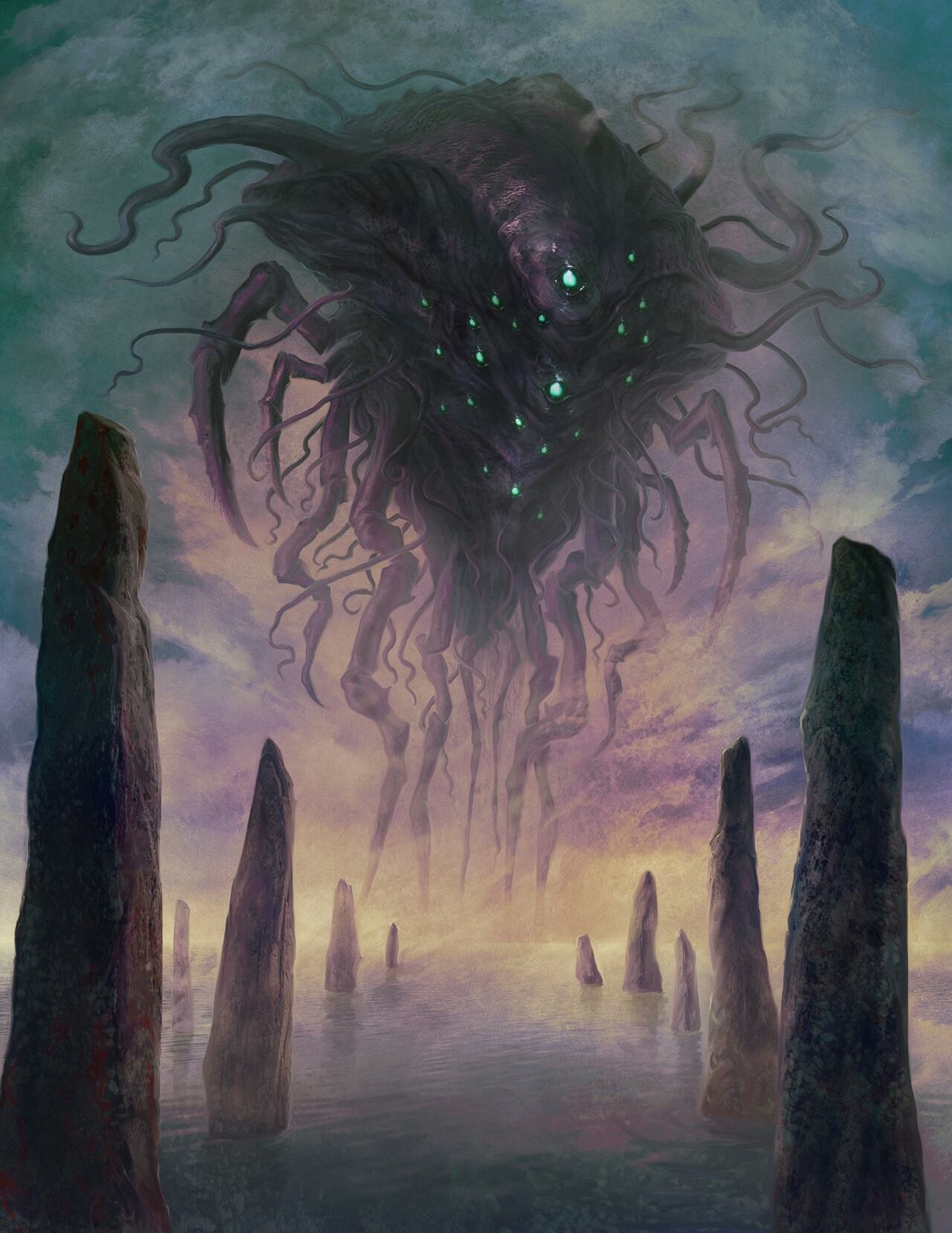"An ethereal, computerized rendering portrays a strikingly surreal landscape reminiscent of a painting. The scene is dominated by a silvery, white body of water occupying the bottom quarter of the image. Emerging from this water are tall, slender standing stones, arranged in two rows flanking the composition—larger and more prominent in the foreground, gradually diminishing in size and height as they recede into the distance. Centered above this watery expanse is a floating, diamond-shaped entity, rendered in shades of gray. This ethereal creature, with numerous tentacles extending upward, sideways, and cascading downwards towards the water, exudes an otherworldly presence. Intriguingly, it is adorned with a scattering of tiny light specks, lending it a mystical glow. The sky above the enigmatic figure transitions from steely gray and blue hues at the top to a vibrant palette of pink and purple below, culminating in a lighter, orange-tinged horizon near the waterline. This dreamlike, fantastical tableau captivates with its intricate details and hauntingly beautiful atmosphere."